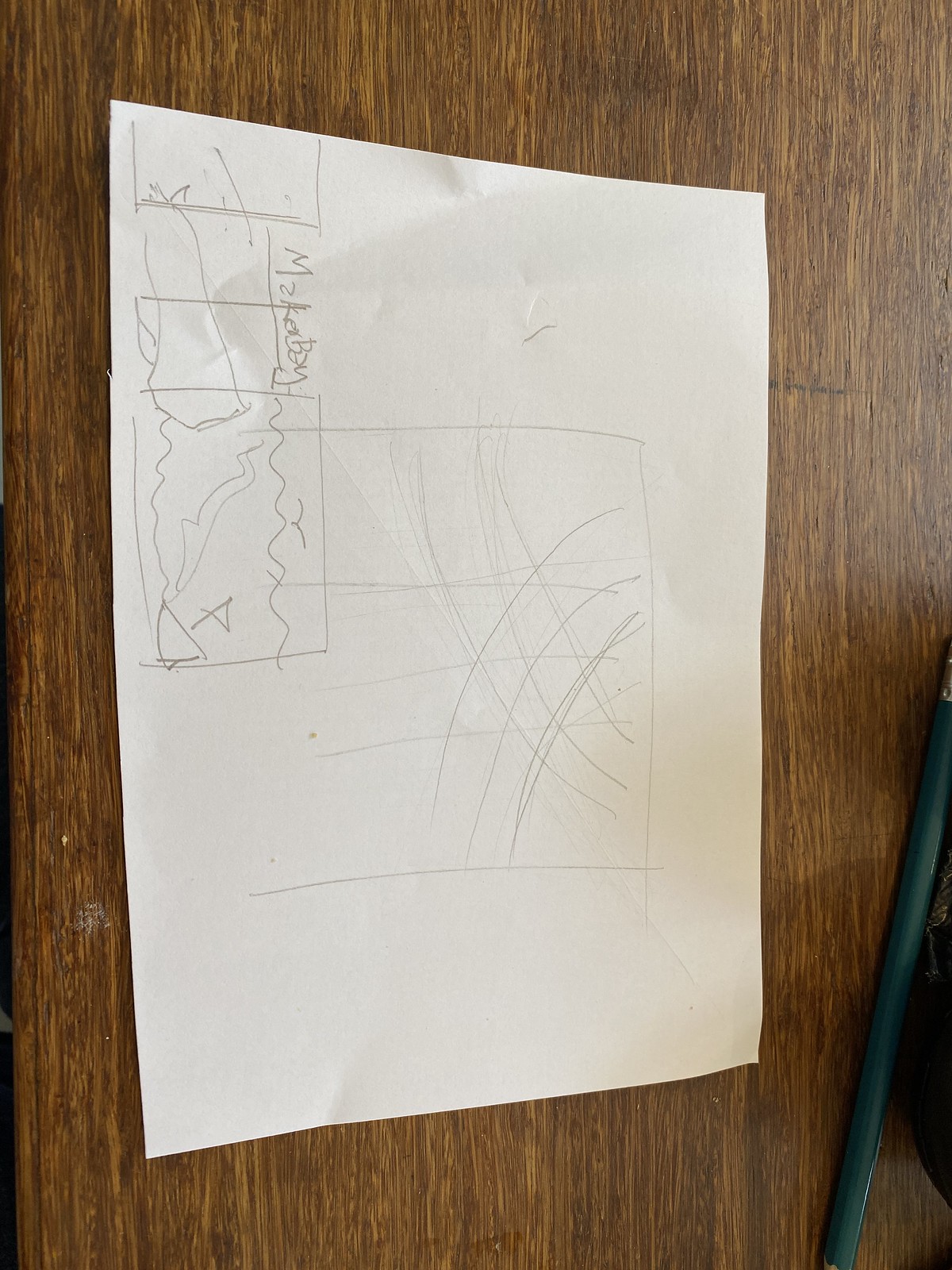The image showcases a detailed, grain-marked wooden panel with a rich brown color accented by lighter streaks. Adhered to the wooden surface is a white piece of paper featuring sketchy, indiscernible drawings that evoke the semblance of maps or preliminary layout plans. The left side of the paper bears a cryptic word starting with a capital 'M' and 'Z', followed by letters that are difficult to identify, suggesting it may not be in a familiar European language. In the left-hand corner of the paper, there is a drawing of a triangle with a small flag, while the right-hand side is filled with interwoven curved lines crossing each other. Adding to the complexity, a grey rod or plastic-coated wire traverses the lower quarter of the wooden background, further contributing to the enigmatic nature of this scene.